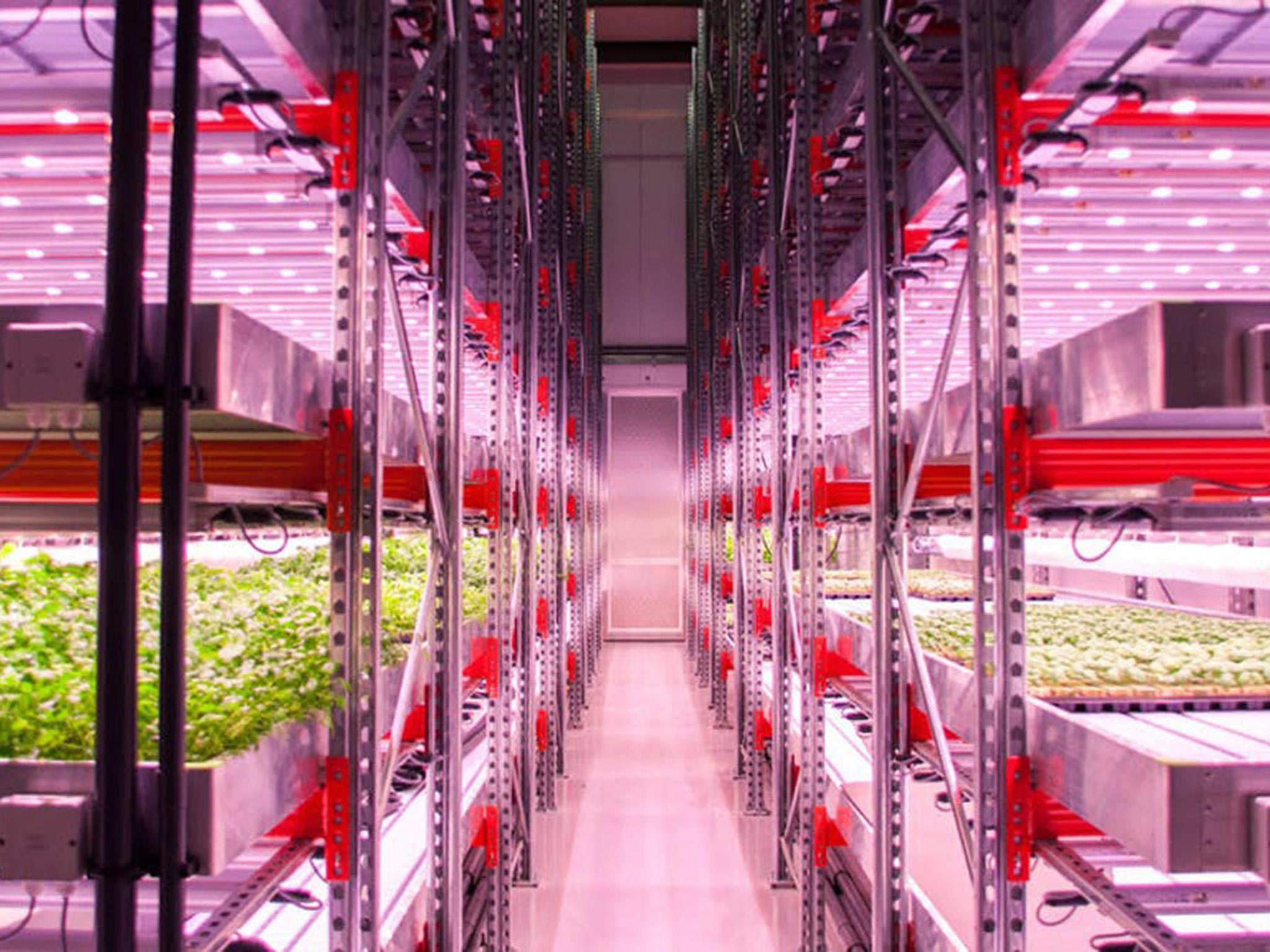The photograph depicts the interior of a plant nursery within a warehouse, featuring an industrial setup with large metal shelving units spanning from the floor to the lofty ceiling. These shelves are arranged along both sides of a central aisle, which serves as the pathway for moving through the space. The shelves are laden with an array of green plants, housed in black plastic containers. On the left side, the plants appear bushier, resembling herbs like cilantro, while the plants on the right are smaller in comparison. The entire scene is bathed in vibrant lighting, which gives a distinctive pinkish hue to the shelving units, door, and surroundings. This vivid illumination is provided by numerous small white lights installed on each shelf, casting a warm, colorful glow that enhances the overall aesthetic of the nursery. Additionally, the underside of each shelf is accentuated with red spots, contributing further to the eye-catching and colorful environment. The photo is devoid of any text or writing, focusing solely on the vivid and orderly presentation of the indoor plant nursery.